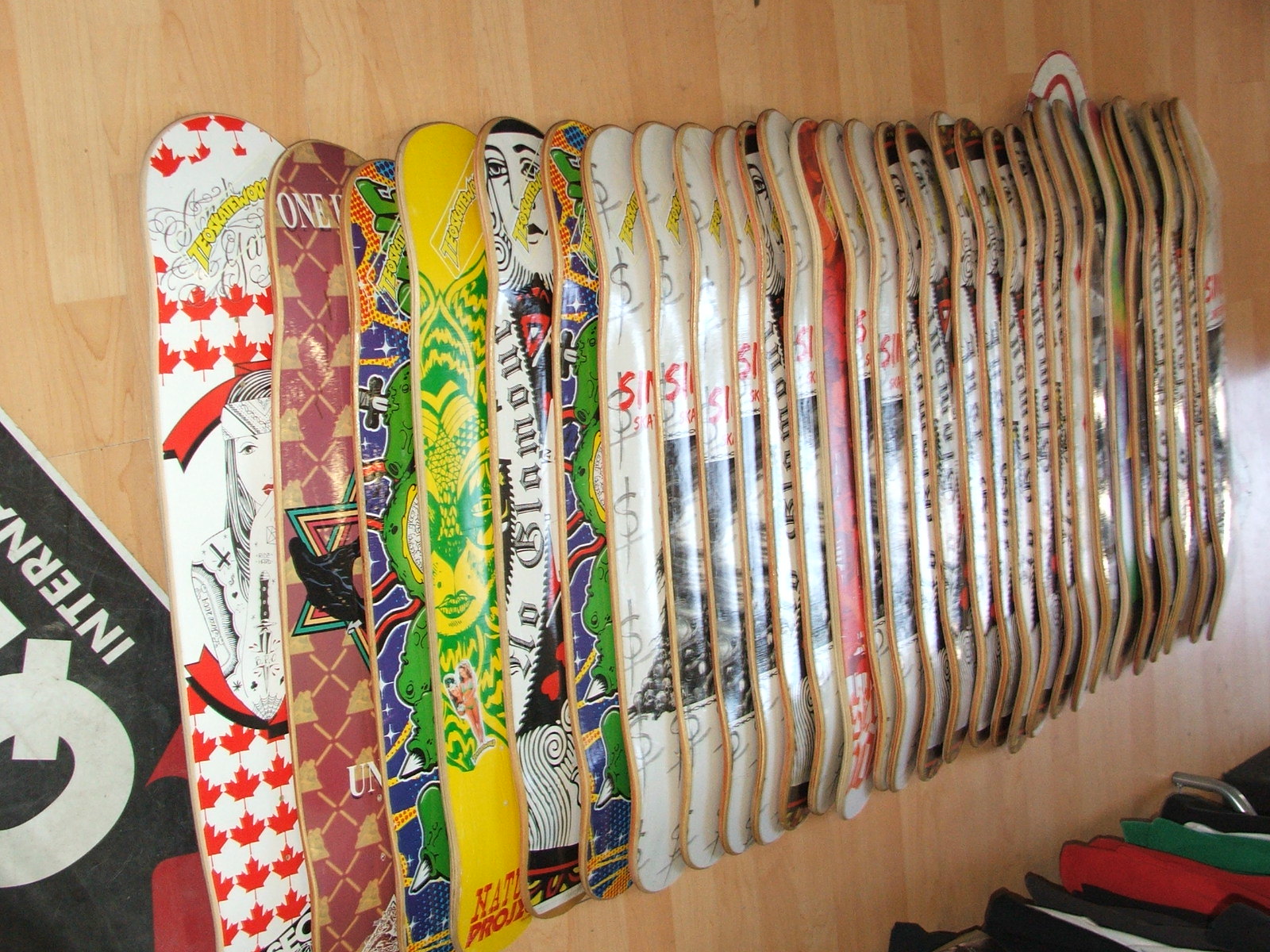This photograph showcases a vibrant collection of approximately 20 skateboards arranged on a light wood floor, although the image's orientation makes it appear almost like a wall. The boards overlap each other, making it difficult to discern individual designs, but their glossy, smooth finishes and colorful patterns are evident. Dominant colors include green, yellow, red, white, black, and blue. Notably, the skateboard on the far right features a repeating Canadian flag design framing a woman's image, while the adjacent board displays a Star of David in green, yellow, and red atop a Louis Vuitton-style background. In the bottom left corner, there is a partially visible black, white, and red poster with the letters "Q" and "Intern" discernible. The bottom right corner reveals a clothing rack with long-sleeve hoodies or sweatshirts in black, white, red, and green hues. The scene is lively, and the skateboards' polished surfaces and intricate designs add to the dynamic visual appeal.